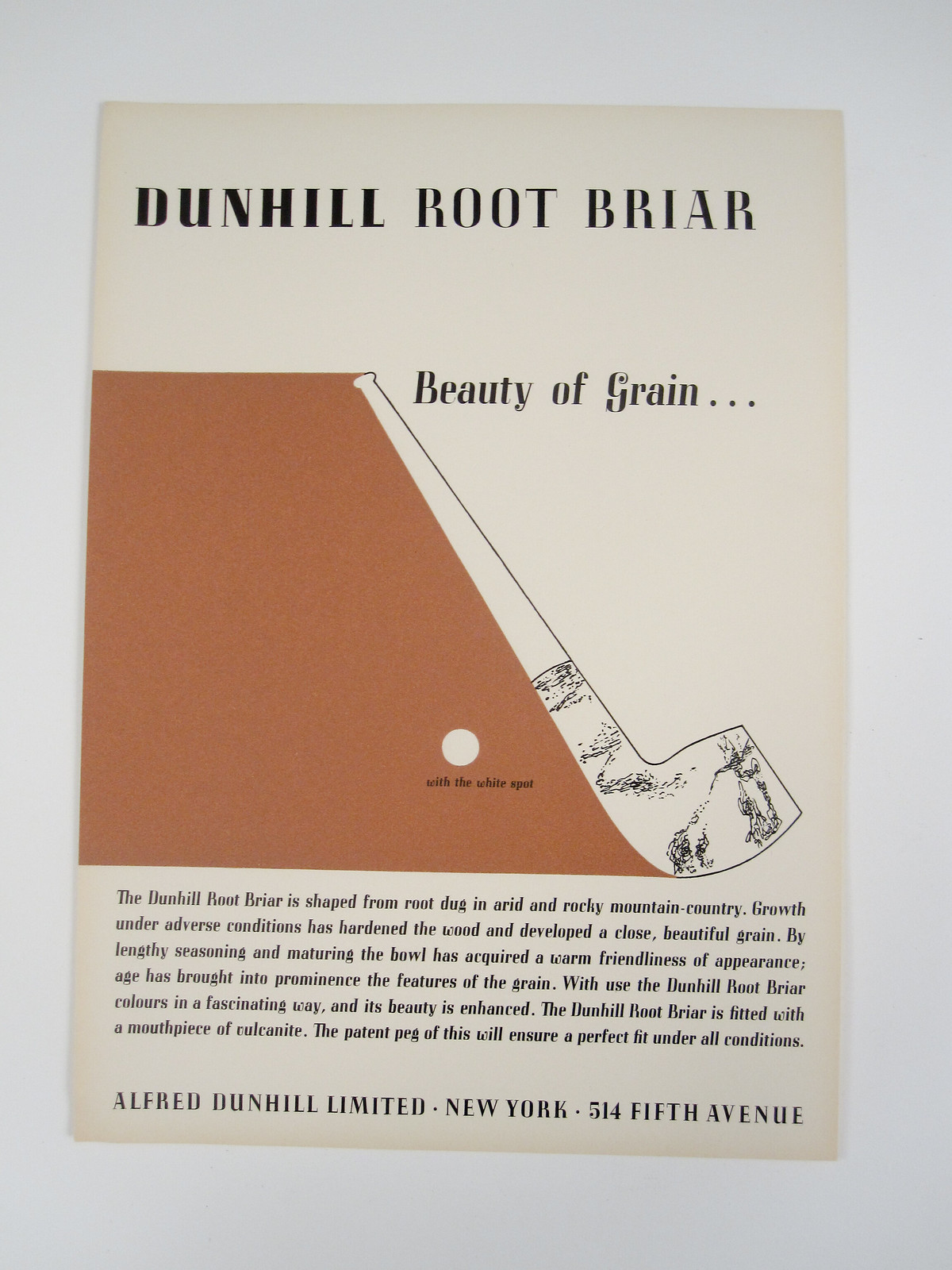The image depicts an advertisement for Dunhill Root Briar, a smoking pipe made by the famous tobacco company Alfred Dunhill Limited. The sheet of paper, beige in color against a whitish background, prominently displays "Dunhill Root Briar" at the top, followed by "Beauty of Grain." To the left, there is a brown trapezoid shape with a white circle inside it, labeled "The White Spot," and on the right, a slightly blurry illustration resembling a pipe with a lacrosse or hockey stick-like shape. Below the illustration, a descriptive paragraph reads:

"The Dunhill Root Briar is shaped from root dug in arid and rocky mountain country. Growth under adverse conditions has hardened the wood and developed a close, beautiful grain. By lengthy seasoning and maturing, the bowl has acquired a warm friendliness of appearance. Age has brought into prominence the features of the grain. With use, the Dunhill Root Briar colors in a fascinating way and its beauty is enhanced. The Dunhill Root Briar is fitted with a mouthpiece of vulcanite. The patent peg of this will ensure a perfect fit under all conditions."

At the bottom, the ad mentions the company’s address: "Alfred Dunhill Limited, New York, 514 5th Avenue."